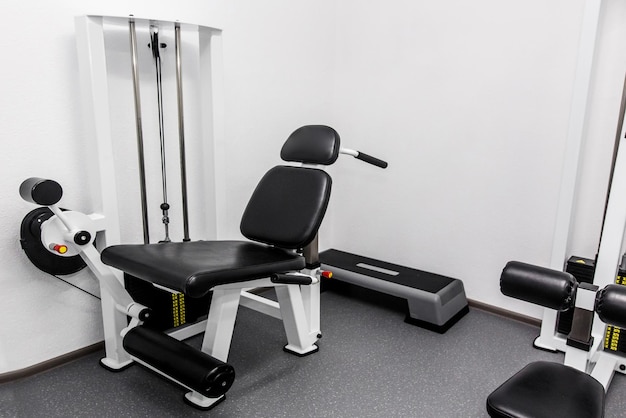The image showcases a small, minimalist personal gym with clean, white walls and a plain gray speckled floor. Central to the scene is a weightlifting machine with black leather upholstery, positioned slightly left of center. This machine features several bars for gripping and various lifting exercises, along with padded areas for leg support, likely for thigh and calf workouts. Adjacent to it, and up against the wall, is a stepper used for step or aerobic exercises.

Behind this primary machine, there's a small stool, also crafted for gym use. To the right, partially cut off in the image, there is another machine with a small seat area and two coated soft panels designed for lifting exercises. The equipment exhibits a sleek and practical design, prominently featuring black seats and white metal rods, creating a modern and organized workout space.